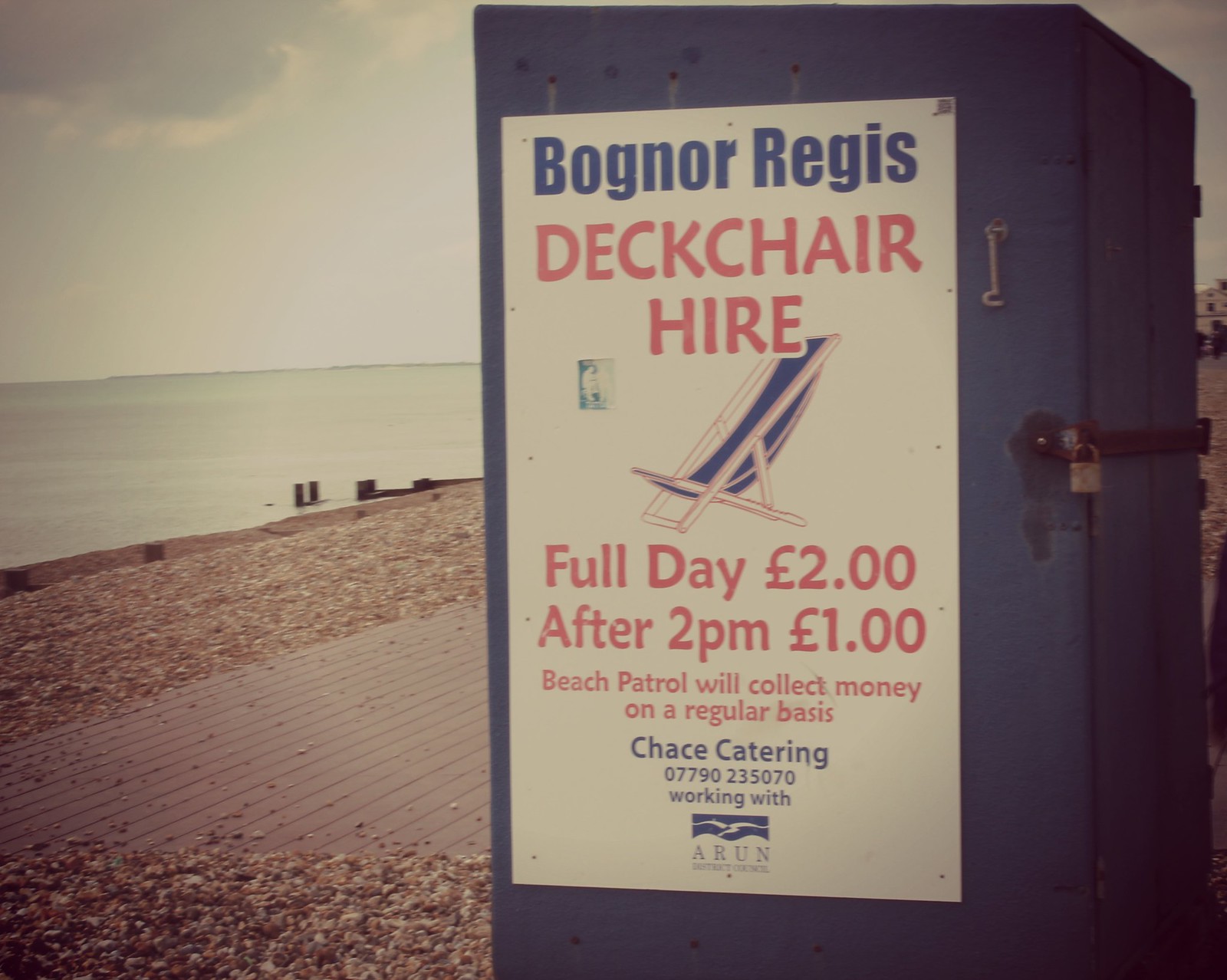The photograph captures an old, weathered, dark blue shed situated near a pebble beach and a boardwalk, possibly during daylight hours. Dominating the right half of the image, the shed is constructed from painted blue metal, showing signs of age with rusted parts securing a large padlocked bar. Above the lock, a small hook is affixed to the shed's side. Prominently displayed on the shed is a white poster with red and blue text, which reads: "Bognor Regis Deck Chair Hire. Full day: two pounds. After 2 p.m.: one pound. Beach Patrol will collect money on a regular basis." The lower section of the poster mentions "Chase Catering 07790-235-070" and features a logo of a white bird on a blue background with the text "ARUN" below it, accompanied by additional, unreadable text. The overall image has a faded, washed-out quality, reminiscent of an old color photograph. In the background to the left, the scene includes a pebble beach and a wooden boardwalk or pier, with water visible further in the distance.